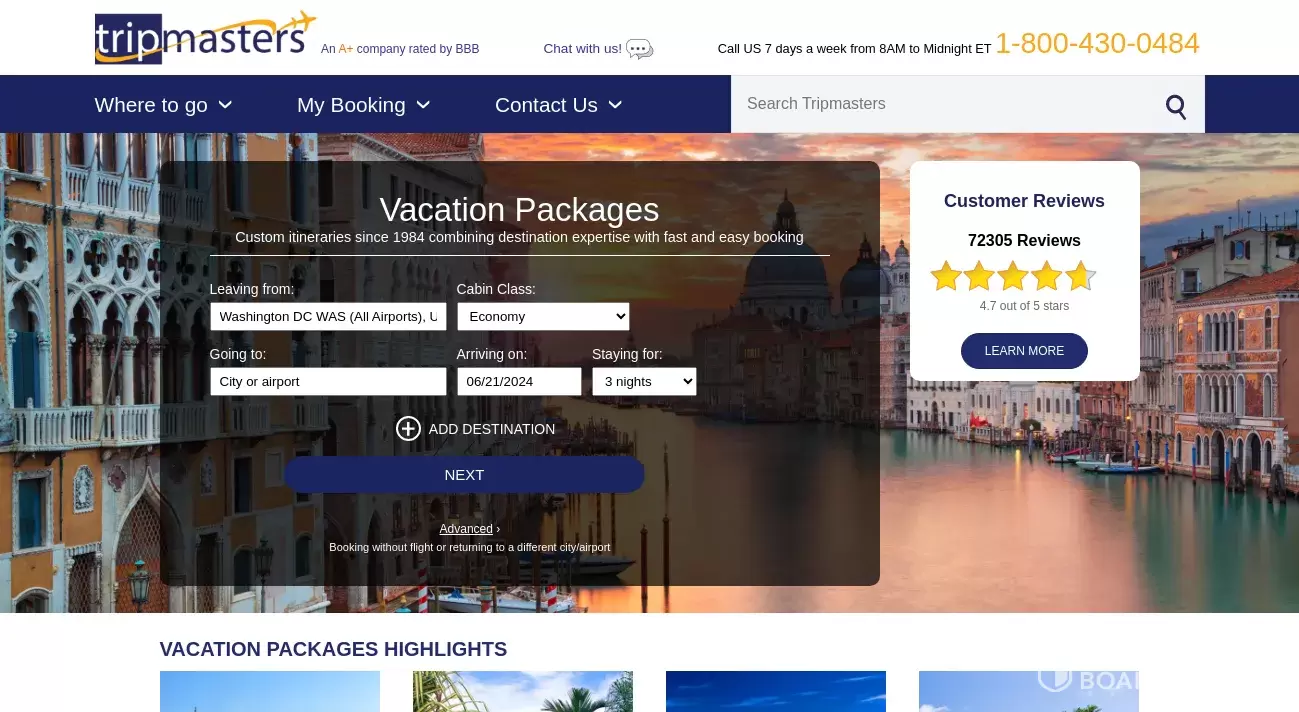Here is a cleaned-up and detailed caption for the described image of the website homepage for Tripmasters:

---

**Tripmasters Homepage Image**

The image displays the homepage of the Tripmasters website. In the upper left corner, the Tripmasters logo is prominently featured, with "Trip" set against a dark blue background and "Masters" in contrasting white. A stylized airplane graphic appears to the right, with its tail end playfully touching the letters 'E' and 'R'.

To the right of the logo, there are several notable elements:
- An A+ rating badge from the Better Business Bureau (BBB).
- A chat option labeled "Chat with us."
- A circled oval icon with three dots.
- A contact prompt stating, "Call us seven days a week from 8 a.m. to midnight ET," followed by a 1-800 number.

The entire top banner is white, providing a crisp and clean look.

Below the top banner, on the left-hand side, there are menu options labeled "Where to go," "My booking," and "Contact us," each accompanied by drop-down arrows. On the right side of this section, a rectangular search bar is labeled "Search Tripmasters" with a magnifying glass icon to its right.

Centered below this header area, the main section features a beautiful background image of Venice, capturing the serene evening atmosphere with its iconic canals and classic architecture. 

Superimposed on this picturesque background is a form for vacation packages, featuring various input fields:
- **Overlands and leaving from:** [Location Input]
- **Going to:** [Destination Input]
- **Arriving on:** [Date Input]
- **Staying for:** [Duration Input]
- An "Add destination" button and a primary action button labeled "Next" to its right.

To the right-hand side of this form, there is a section showcasing customer reviews, featuring a rating of 4.7 out of 5 stars and a "Learn more" button below the rating.

---

This detailed caption provides a clear and comprehensive description of the Tripmasters homepage, ensuring that readers can visualize the layout and key components of the webpage.